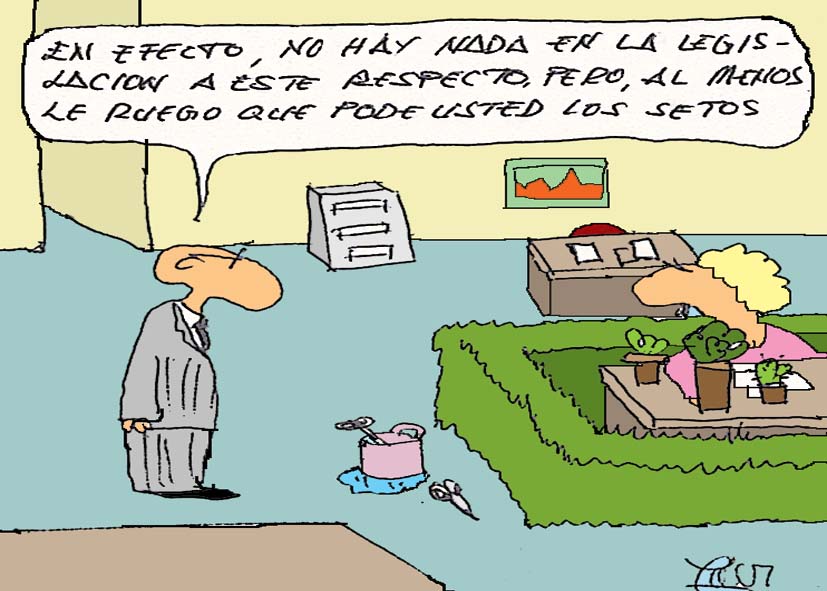In this cartoon image, set within an office environment featuring blue floors and beige walls, a bald, older man with glasses and dressed in a frumpy gray suit stands with a speech bubble above his head. The bubble contains Spanish text: "En efecto no hay nada en la legislación Este respecto pero al menos la ruego que puede usted los cetos," which translates to "Indeed, there is nothing in the legislation in this regard, but at least I beg you to put down the hedges." The man's head humorously resembles a peanut from the side. Opposite him, a blonde woman sits at a desk, which is uniquely surrounded by neatly trimmed hedges, forming a square around her workstation. Additional details include a pair of scissors discarded in a garbage can and a painting hanging on the wall behind the woman.